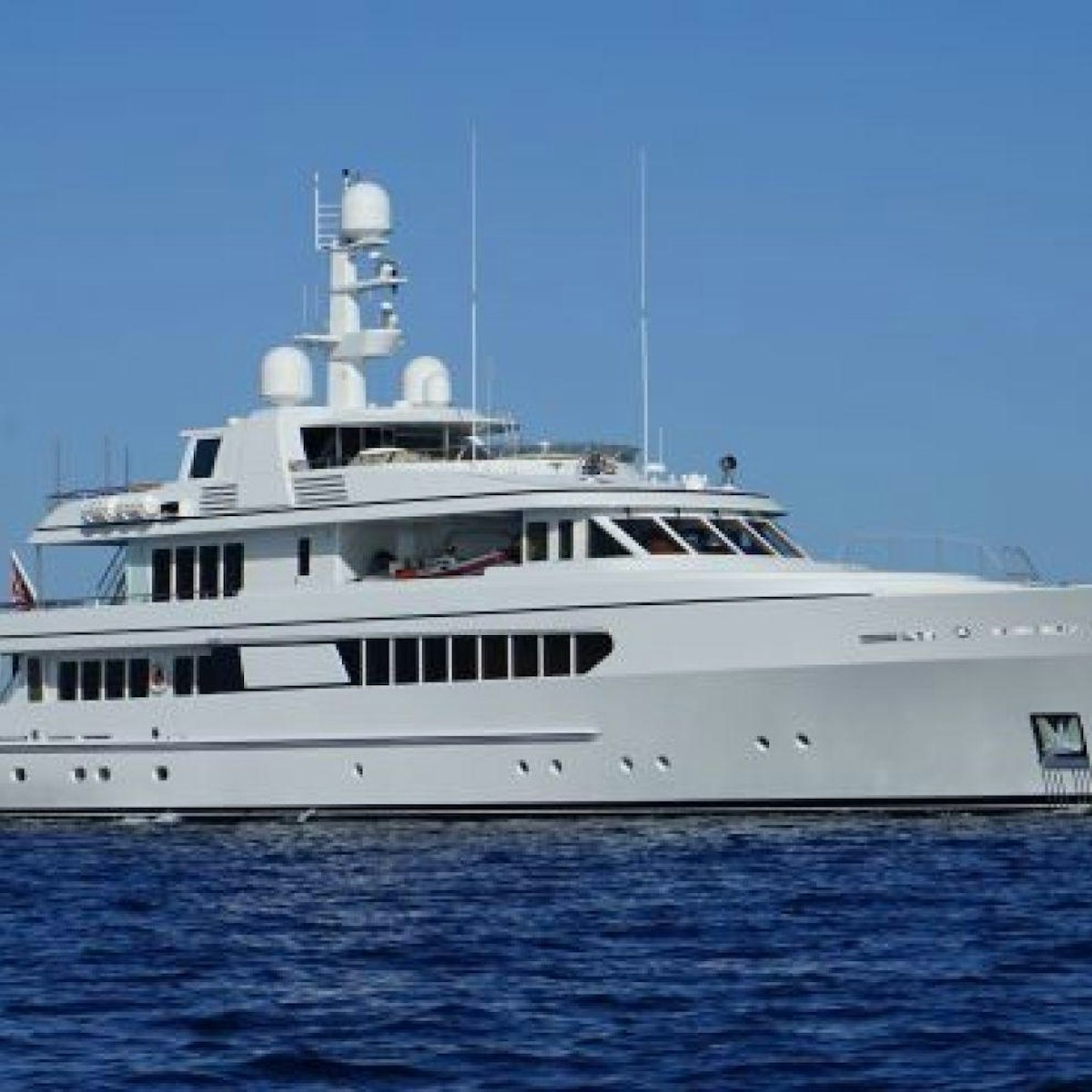This photograph captures a massive, white yacht positioned centrally in the frame, so large that neither the bow nor the stern is visible. The vessel, likely a yacht, features three levels adorned with sleek, blackout windows. Atop, there are various pieces of equipment, including poles and rounded white structures, possibly for communication and weather monitoring. The yacht sails—or possibly idles—on an extraordinarily deep blue ocean, almost navy in hue, with only gentle ripples marring its surface. There's no indication of any activity on board as no people are visible and there are no discernible names or markings save for a wing-like symbol on the right side. The backdrop is a flawless, cloudless sky, its bright blue complementing the darker tones of the water below. The overall scene conveys a serene, calm day at sea.